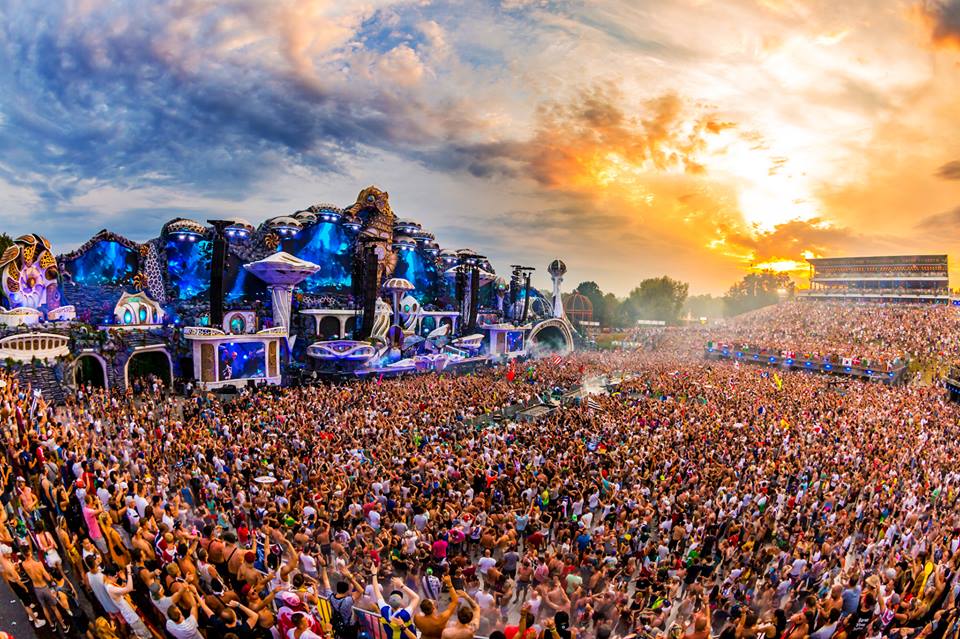The image is a highly detailed drawing or painting of an immense crowd gathered in a stadium-like setting as the sun sets. The sheer number of people is staggering, creating a sea of faces and raised arms that nearly covers the entire ground. They surround a central dark blue structure adorned with white accents, emanating an otherworldly appearance reminiscent of something out of Willy Wonka or an amusement park. This building features a prominent dark brown piece sticking up in the middle, possibly a stage, which is the tallest element in the composition. In front of it, whimsical white mushroom or umbrella-shaped structures add to the surreal atmosphere. Further in the background, grandstands brimming with more people stretch into the distance. On the left, flanking the building, there are homes or smaller structures, while to the right, trees frame the scene. The sky above is a swirling mix of blue, orange, and yellow hues, with the sun dipping below the horizon, casting a magical glow over the entire scene. The combination of the crowded setting and fantastical architecture makes the scene almost unbelievable, blurring the line between reality and imagination.